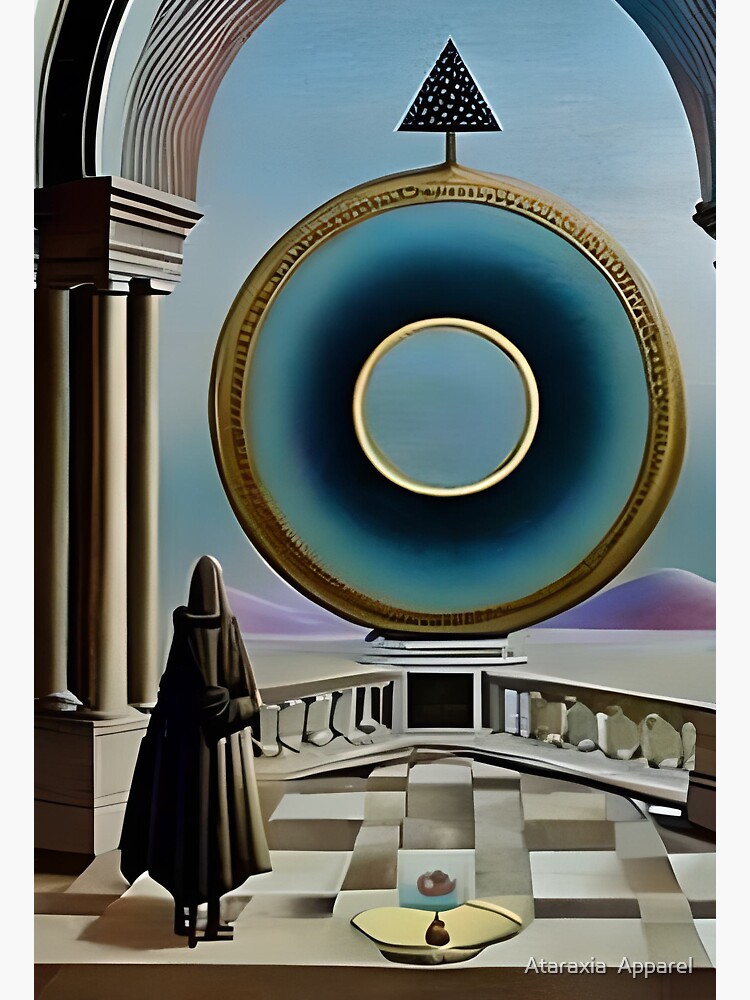This image appears to be a highly detailed, futuristic art poster bordered in white, which bears a caption at the bottom right reading "Atorexia Apparel." The scene captures a fantastical, sci-fi setting featuring a richly textured balcony constructed from marble with balusters, tall white columns, and intricate arches overhead. The floor below is patterned in grays and browns, resembling a checkerboard with a raised center, and a small gold pool with brown and blue hues adorns the bottom center.

A central figure clad in a long brown cloak and a brown headdress or hood stands on this balcony. The figure has arms crossed, and their features are obscured, adding an air of mystery. The balcony extends out towards a breathtaking landscape, where purple mountains stretch across the horizon. Dominating the scene in the distance is a colossal ring, outlined in gold, which transitions from light blue at its edges to dark blue at its center. This ring features a gold-lined hole and has a stylized black triangle with intricate etchings at the top.

The harmonious blend of classical architectural elements with otherworldly features and colors creates a compelling contrast, enhancing the sci-fi fantasy ambiance of the illustration.